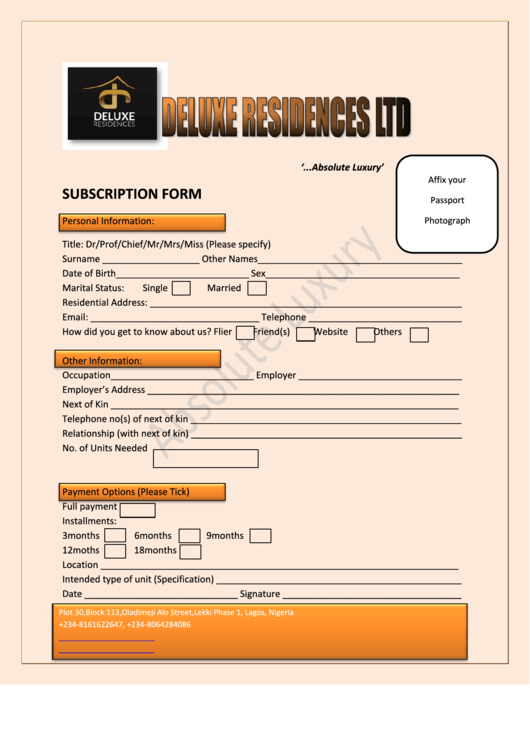This image features a detailed subscription form for Deluxe Residences Limited. The form is presented on a rectangular light pink sheet of paper with a gold thin border encompassing the entire perimeter. In the upper left-hand corner, there is a solid black square logo with a gold image inside, and beneath in white uppercase letters, it reads "DELUXE." To the right of the logo, "DELUXE RESIDENCES LTD" is emblazoned in large gold capital letters. 

The form is meticulously sectioned, starting with a header in black capital letters that reads "SUBSCRIPTION FORM." Below this, an orange rectangle labeled "PERSONAL INFORMATION" outlines several lines for input: title selection, surname, date of birth, marital status, residential address, email, and how the individual became aware of the company. 

Further down, another orange rectangle labeled "OTHER INFORMATION" asks for details such as occupation, employer's address, next of kin, telephone number, relationship, and the number of units required. 

The last section, marked by an orange rectangle labeled "PAYMENT OPTIONS (please tick)," provides choices for full payment or installment plans, along with sections for specifying the location, intended type of unit, and a spot for the date. 

Additionally, there's a designated area at the top for attaching a passport photo, enhancing the comprehensiveness of the form.